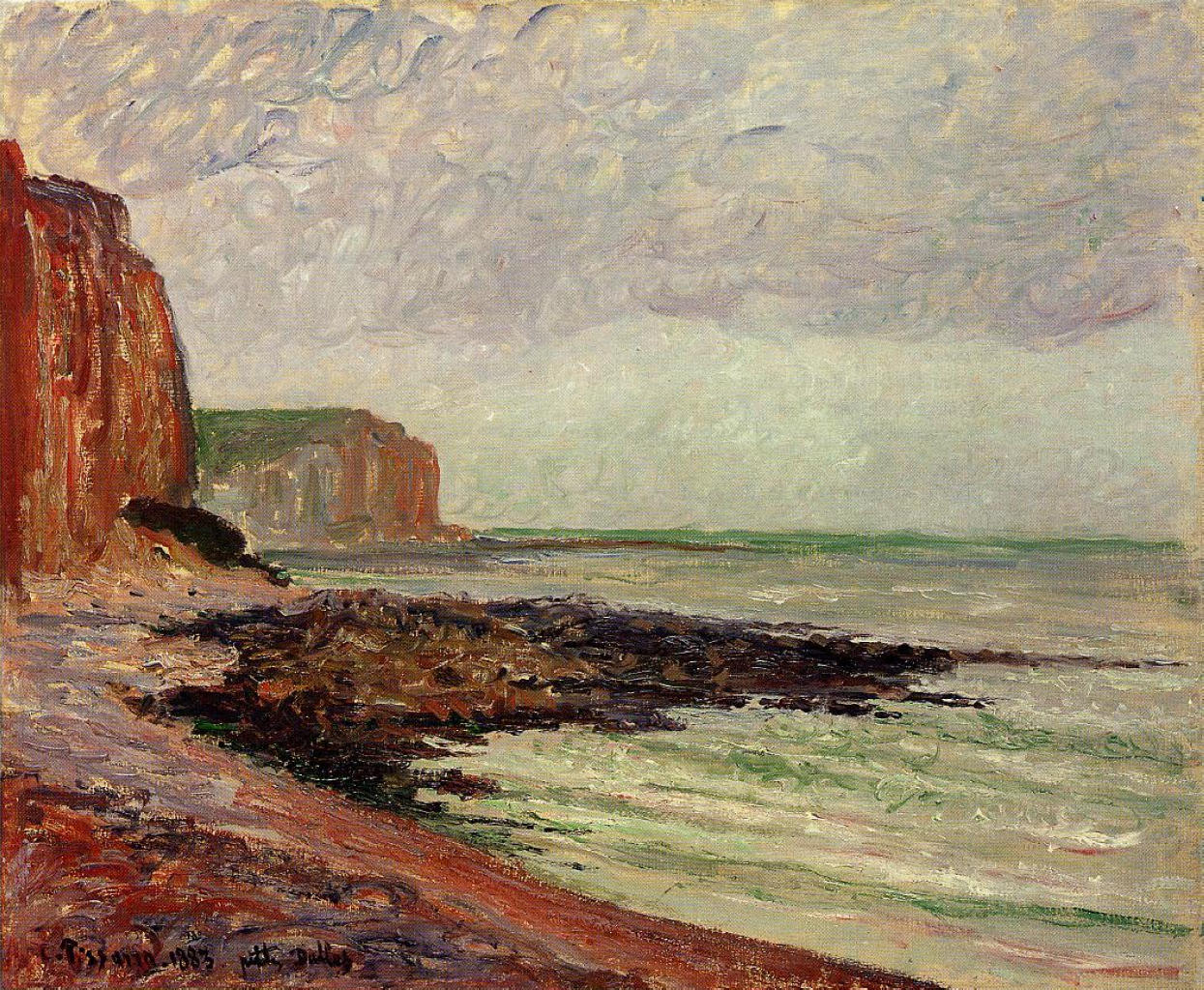This detailed impressionistic watercolor painting from 1883 captures a striking coastal scene featuring tall, reddish-brown cliffs on the left foreground and a faded cliff in the background. The cliffs blend into the beach, which shares the same reddish hues, and a rocky jetty juts out into the light seafoam green water on the right. The sky is depicted with loose, scribbly circles suggesting soft gray clouds against a light blue-gray backdrop. The shoreline bends into the distance, leading the viewer's eye along the horizon. The artist's signature, starting with a 'P' and accompanied by the date 1883, is located in the bottom left corner, though parts of the inscription are difficult to decipher. No people or additional objects disturb the serene landscape, emphasizing the natural beauty of the coastline.